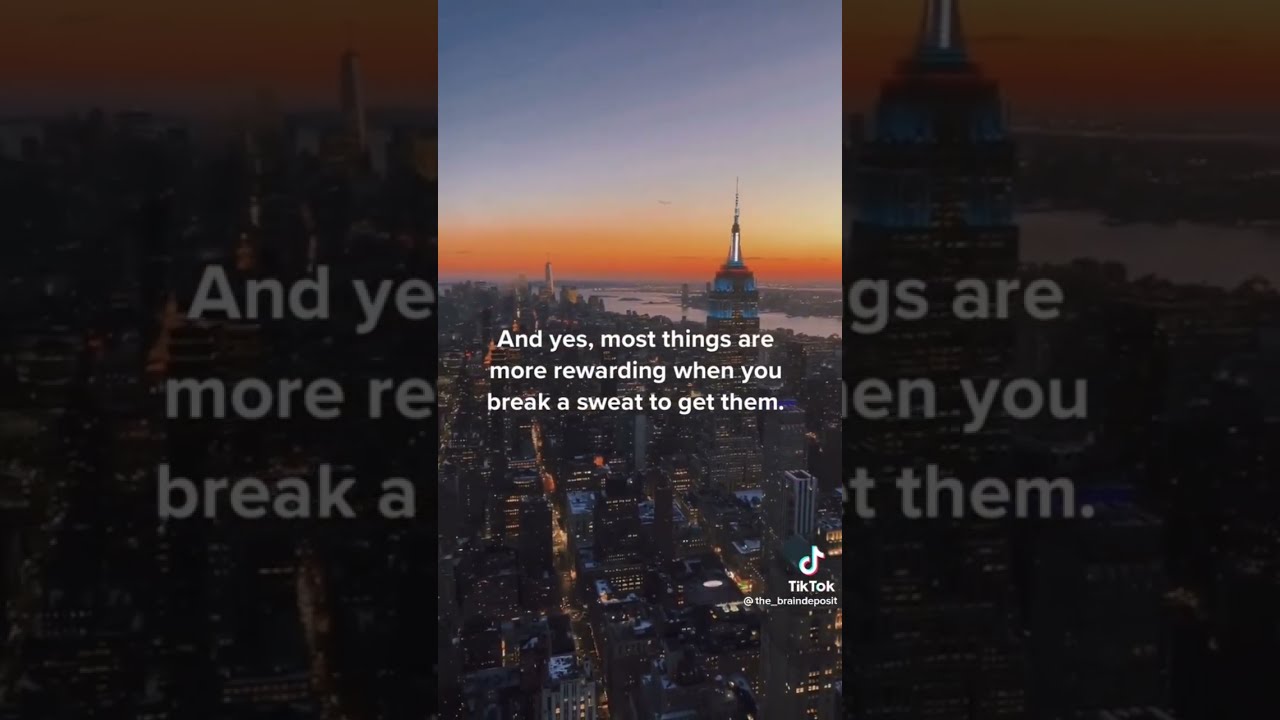The image is a still shot from a TikTok video featuring a striking bird's-eye view of a bustling cityscape, likely New York City, considering the dense arrangement of buildings and the presence of what could be the Empire State Building. The photo, captured in portrait orientation, includes partial, fragmented images on the left and right sides. Dominating the background is a picturesque sunset, progressing from deep blue at the top of the sky to vibrant oranges and reds near the horizon, casting a soft glow over the city. Prominently displayed across the middle of the image is the motivational text: "And yes, most things are more rewarding when you break a sweat to get them." The TikTok logo is visible in the bottom right corner, confirming the platform it was shared on.